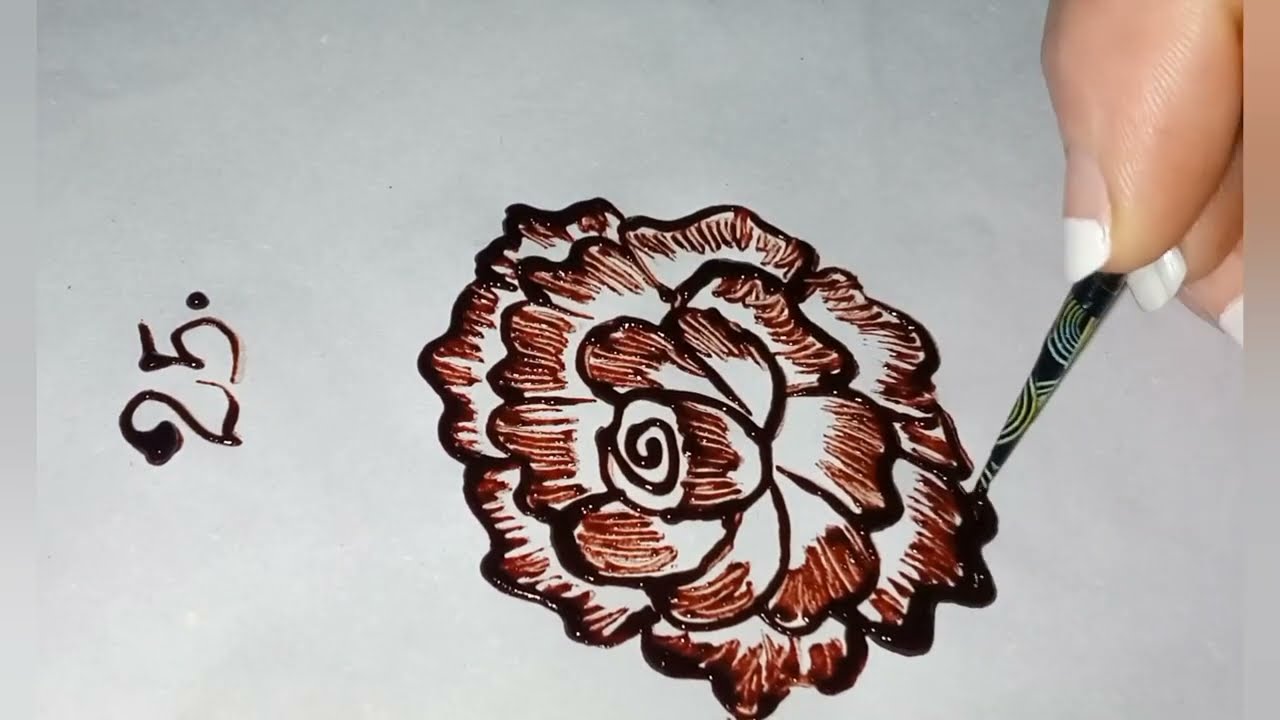In the image, a woman with French-manicured nails is captured in the midst of painting. The scene is set against a stark white background. Her hand, adorned with a black paintbrush featuring intricate white patterns, enters the frame from the top right corner. The focus of her artistry is a detailed, close-up depiction of a rose. The rose is characterized by its open petals, with the center intricately curled and surrounded by concentric rows of larger petals. The petals exhibit shaded brown lines, adding texture and dimension to the flower. The entire rose is outlined in black, creating a sharp contrast against the background. Notably, the image includes a number "25." The digits are vertically oriented, with a thick blotch of paint subtly altering the form of the number “2,” followed by a period. The paint used appears thick and textured, resembling melted chocolate, which adds a sense of depth and a slightly uneven tone to the artwork.